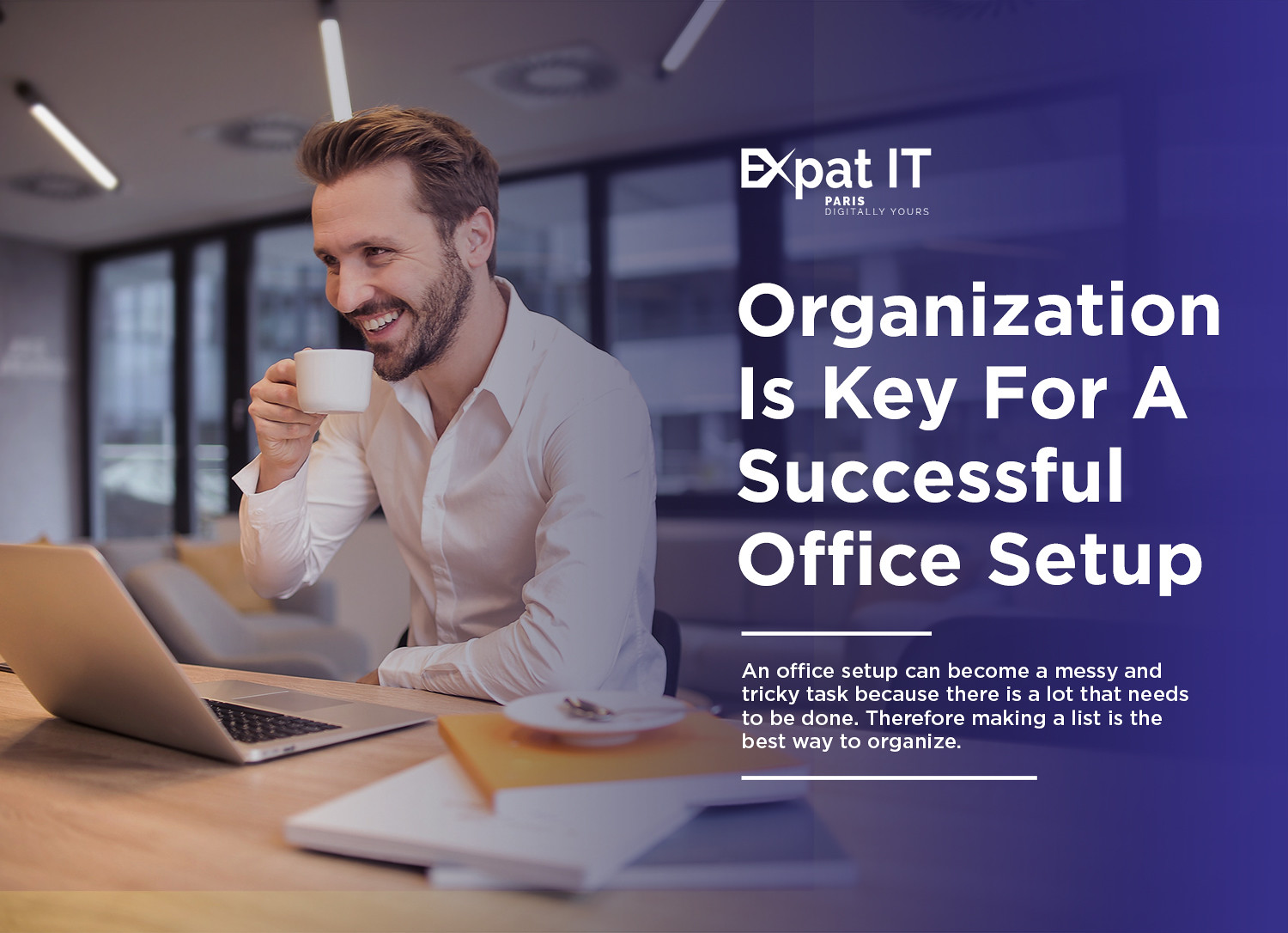This detailed image is a horizontally rectangular poster for the company expat IT, based in Paris. On the left side of the poster, a professionally dressed man in a neatly trimmed beard and white shirt sits at a natural light wooden desk. He is in an office with a professional finish, featuring fluorescent lights and a window in the background. The man holds a coffee cup mid-sip, smiling as if in a meeting, with an open laptop and a plate with a spoon beside it on the desk. The desk is well-organized, displaying neatly arranged books in orange, white, and blue.

The right side of the image transitions into a dark blue and purple background with large white text overlay. The text reads "expat IT Paris" and emphasizes the slogan "Organization is key for a successful office setup." A paragraph below elaborates, stating that "an office setup can become a messy and tricky task because there's a lot that needs to be done; therefore, making a list is the best way to organize." The overall design suggests the poster is an advertisement that highlights the importance of an organized work environment, potentially offering services to assist with office setups.